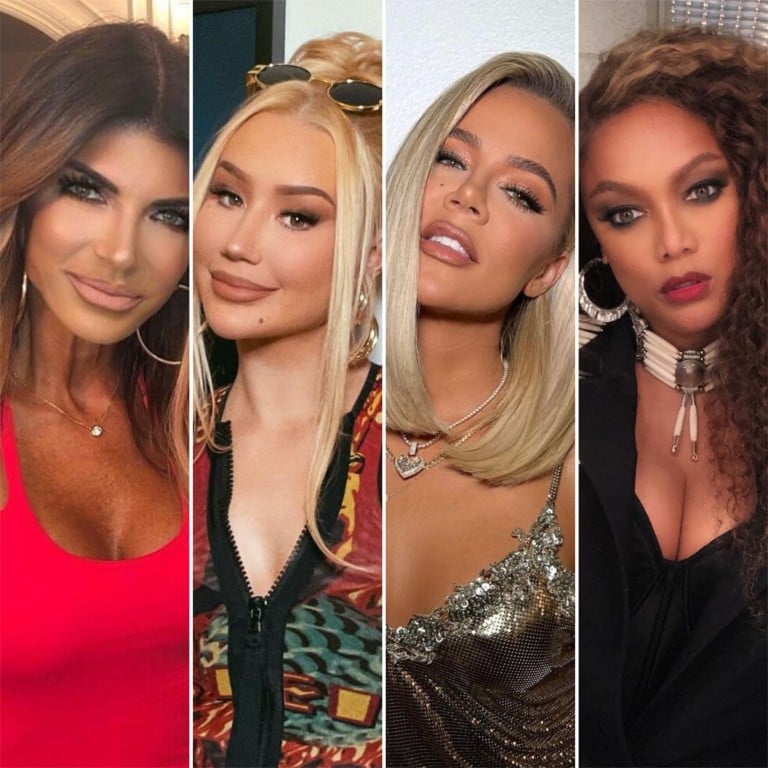This image is a single square compilation of four vertically aligned skinny rectangles, each featuring a famous woman in a close-up shot. The first woman, possibly a Real Housewife, has dark brown hair, prominent fake eyelashes, dark eyebrows, hoop earrings, and a gold necklace. She wears a tight red tank top showcasing her tanned chest, which contrasts with her lighter face. The second woman, a blonde, sports sunglasses on top of her head, some hair pulled up while long pieces hang down. She is adorned with fake eyelashes and makeup and wears an unzipped colorful jacket revealing part of her chest. The third woman, resembling Khloe Kardashian, has blonde hair just past her shoulders, accessorized with necklaces and a sparkling silver tank top. She wears notable makeup and fake eyelashes. The fourth and final woman, possibly Tyra Banks, has curly hair, a striking red lipstick, heavy eye makeup, hoop earrings, and a chunky necklace. She wears a black top with a V-neck that reveals some cleavage. All the women are heavily made-up, and their outfits are stylish and eye-catching, with each image showcasing a different personality through vibrant and detailed presentation, suggesting a possible advertisement.